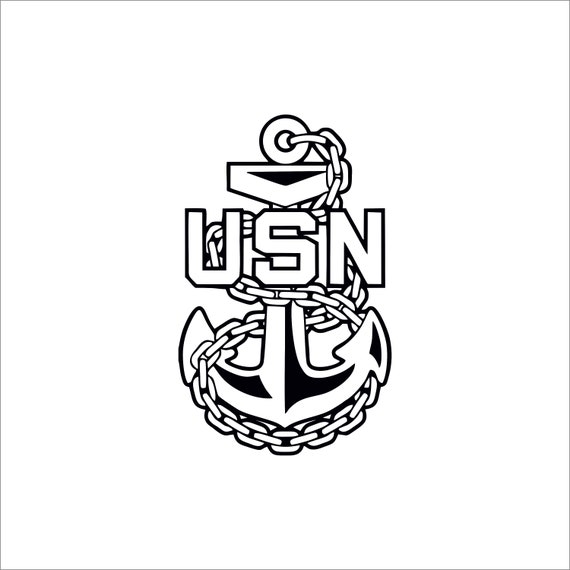This is a black-and-white illustration, likely a sketch designed for a tattoo, featuring a detailed depiction of a logo for the United States Navy. The entire image is framed within a thin black outline, forming a square roughly around 5 or 6 inches by 5 or 6 inches. Dominating the illustration is a large, ship-style anchor, characterized by pointed tips on either side and a crescent shape at the bottom. At the top of the anchor is a dark, upside-down triangle with spiky details on the sides, shaded to give depth. A substantial, heavy chain snakes around the anchor, looping around the top where it connects to a bail or hanging loop that resembles a metal donut. Prominently overlaid on the anchor are the bold black letters "USN," standing for United States Navy, outlined in black with a white fill. The background remains completely white, emphasizing the strong black outlines and solid shading of the illustration.